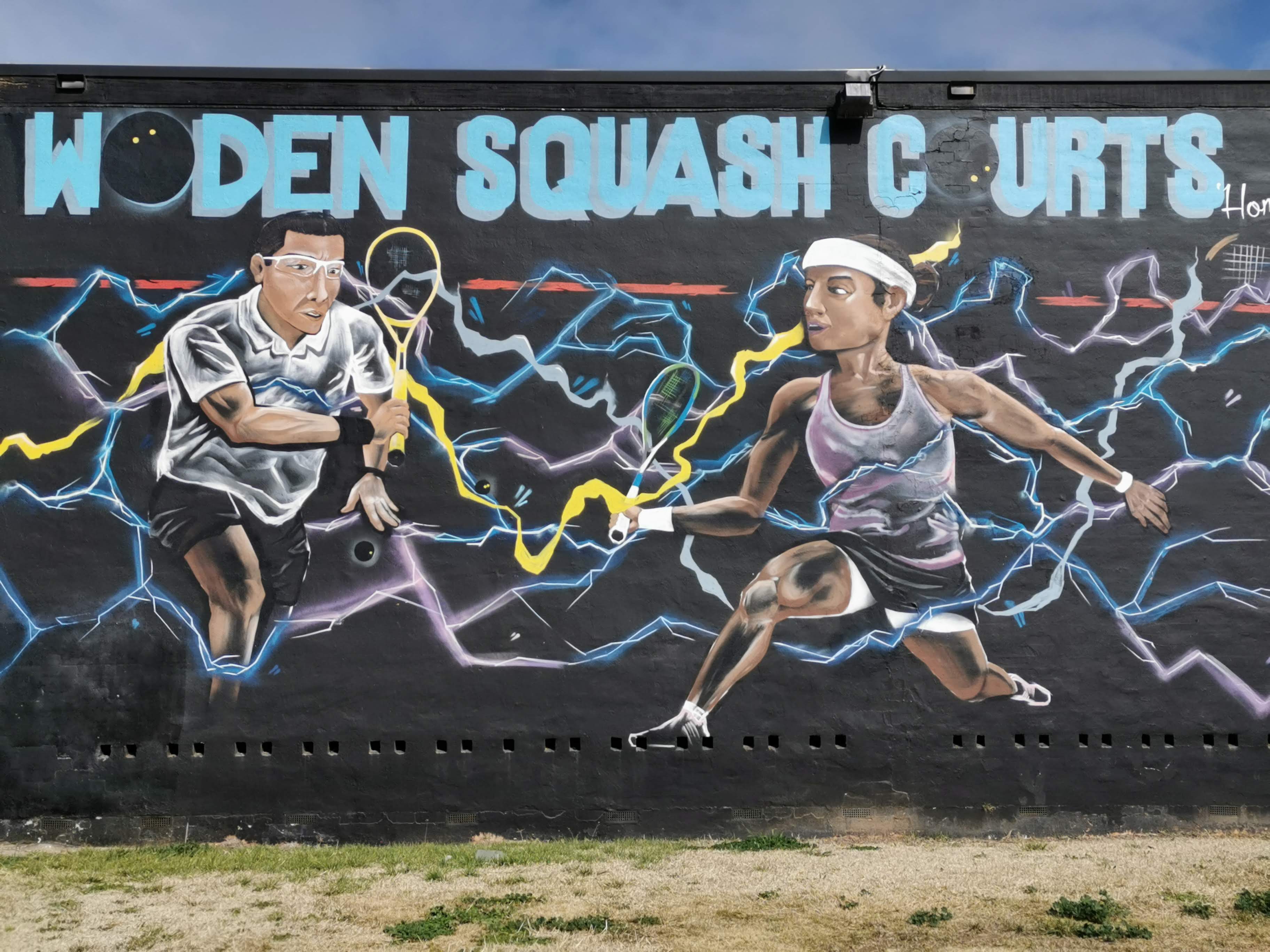The image captures a vibrant outdoor mural painted on a black wall under a bright blue sky with scattered white clouds. The mural prominently features two African-American figures intensely engaged in a squash game, with the words "Woden Squash Courts" emblazoned in blue at the top. 

On the left, there is a male figure clad in a white short-sleeved shirt and black shorts, energetically swinging a vivid yellow squash racket. The man, wearing white glasses, displays a serious and focused demeanor as if in pursuit of the ball. On the right stands a female figure, outfitted in a pink shirt and a white bandana, brandishing a bluish-green squash racket. She shares the same intense focus as her counterpart, emphasizing the competitive nature of their game.

The mural is electrified with colorful lightning bolts, including shades of blue, purple, pink, white, and yellow, making it appear as if energy is radiating from their movements. Below the wall, patches of dead and live grass in varying shades of green and brown can be seen, grounding the mural in its outdoor setting. The overall composition suggests a dynamic and energetic atmosphere, vividly bringing the game and its players to life.